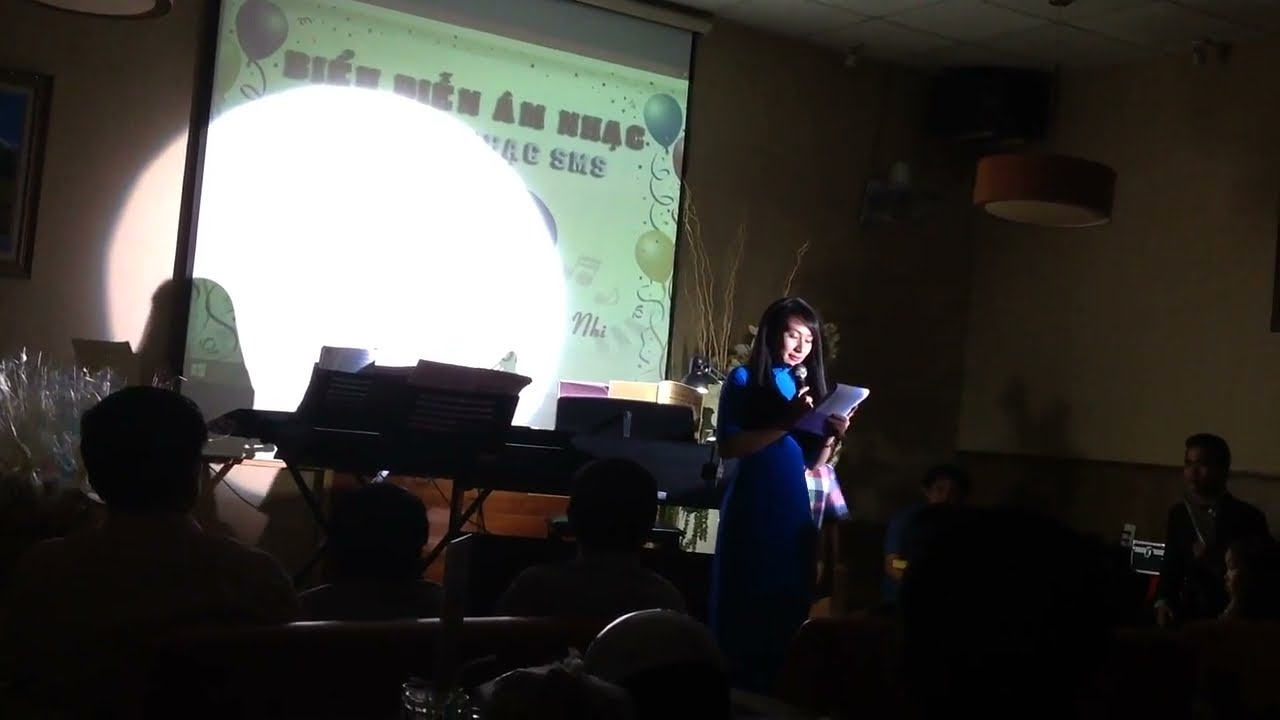The photograph captures an indoor setting in a large, dimly lit room. Dominating the front wall is a display screen projecting an image featuring balloons, an array of text, and a prominent white circle of light. Positioned in the foreground is a table supporting various instruments, papers, and a lamp. Behind this table, partially obscured, sits a person—only the top of their head is visible above the music sheet, suggesting they are at a piano or keyboard, which appears to be deep purple. To the right corner of the table, a person in a blue shirt is seated. Scattered heads of other individuals are seen at the bottom of the image, their backs turned as they attentively face the display. The walls might have a green hue with blue balloons, and the decor includes white flowers and possibly a wall hanging, all bathed in a soft spotlight emanating from the wall. The room's dark ambiance makes it challenging to determine the floor's color or the time of day outside.